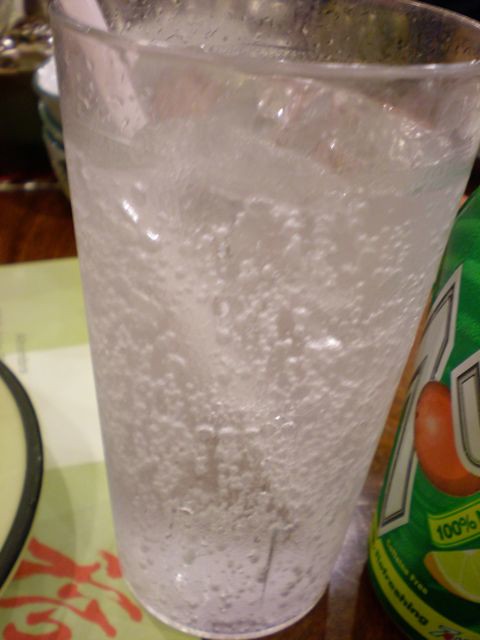The image is a colour, slightly out-of-focus, low-quality, close-up photograph taken indoors, likely on a smartphone, in portrait orientation. It focuses on a clear glass filled with a bubbly liquid, likely 7-Up, with a white straw extending from the bottom right to the top left of the glass. Positioned in the bottom right corner of the photograph is a 7-Up can, partially visible with its distinctive green background, white text outlining a '7', a red cartoon apple or cherry, and part of the letter 'U'. In the background, towards the left, a stack of three bowls can be spotted, the top one being white, obscuring the details of the middle one, and the bottom one displaying a yellow rim. The scene appears to be set on a wooden table, possibly dark oak, partly covered by a lime green placemat featuring an orange or red Japanese symbol. An additional white or cream-colored placemat is visible beneath the glass. The setting suggests a public dining area, likely a restaurant.